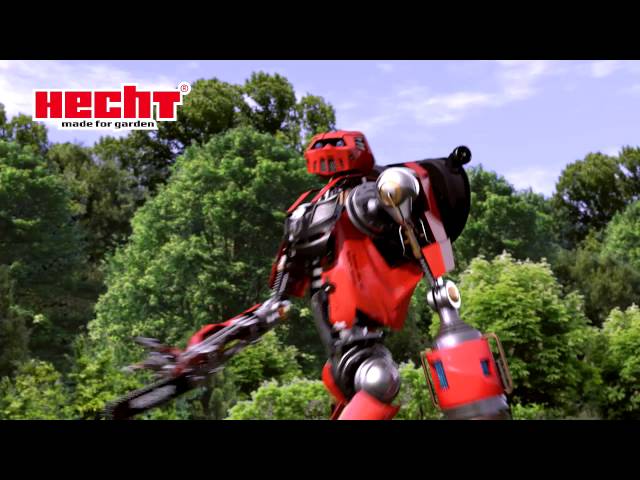The image is a digitally manipulated, slightly blurry screenshot from a video clip featuring a tall, red and silver robot that resembles a transformer walking outdoors. The scene is set against a backdrop of realistic, lush green trees and a bright blue sky with wispy clouds. The robot, prominently positioned in the center, has a red body with silver accents, a head comparable to a cheese grater, and carries a leaf blower while sporting a chainsaw for a right arm. The robot is moving through the forest, seemingly in search of something, with an aggressive demeanor. The video has a thick black border at the top and bottom, and in the top left corner, there is text reading "Hecht" in red, followed by "Made for garden" in black below it.